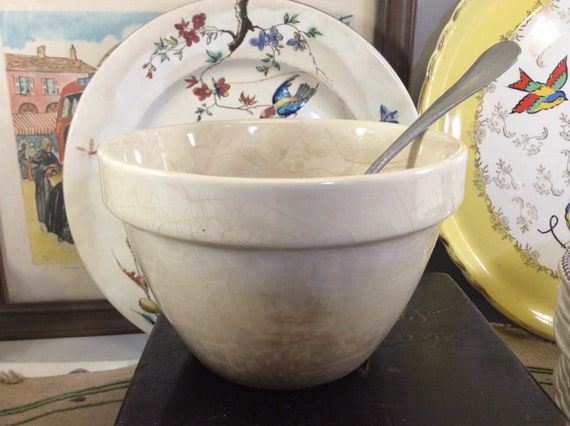In this photograph, a white porcelain bowl with a creamy, off-white tone sits prominently in the foreground. The bowl appears slightly used or dirty and contains a metal utensil, the head of which is not visible, leaving its exact type indeterminate. The bowl rests on a black book, which is placed atop a tablecloth.

Behind the bowl, there are two ceramic plates. The nearer plate showcases intricate artwork featuring flowers and detailed illustrations of old-style Americana birds, which are reminiscent of traditional tattoo designs. The second plate, positioned to the right, is gold-colored and also depicts one of these Americana birds, though with less detail. Partially obscured by these plates is a framed painting, which hints at the image of a pink house. The setting combines elements of rustic charm and vintage artistry, creating an evocative and layered composition.